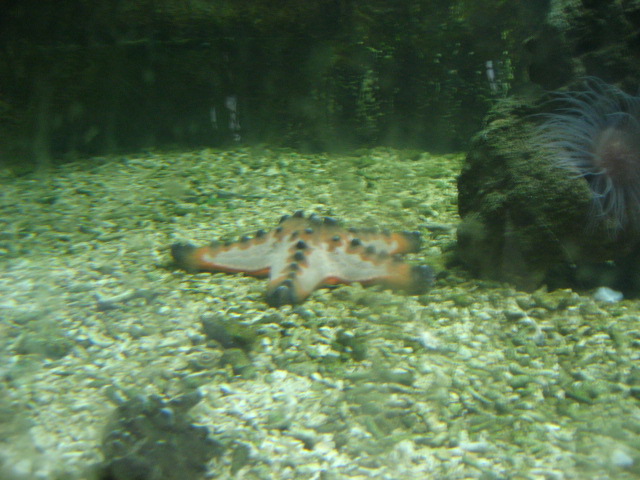This slightly blurry underwater photograph, likely taken in an aquarium or a fish tank, captures the detailed scene at the bottom filled with various marine elements. The image is tinted green due to the water. At the center of the frame lies a starfish, positioned face down on a bed of round, white pebbles. The starfish features an intricate pattern of colors: its body boasts a solid white with orange zigzag lines, transitioning to darker grayish or black tips adorned with black dots and bluer green bumps along the ridges. To the right, a sea anemone with a reddish body and bluish-purple tentacles is attached to a rock, which appears green, likely covered with algae. The background reveals additional greenish seaweed or algae.